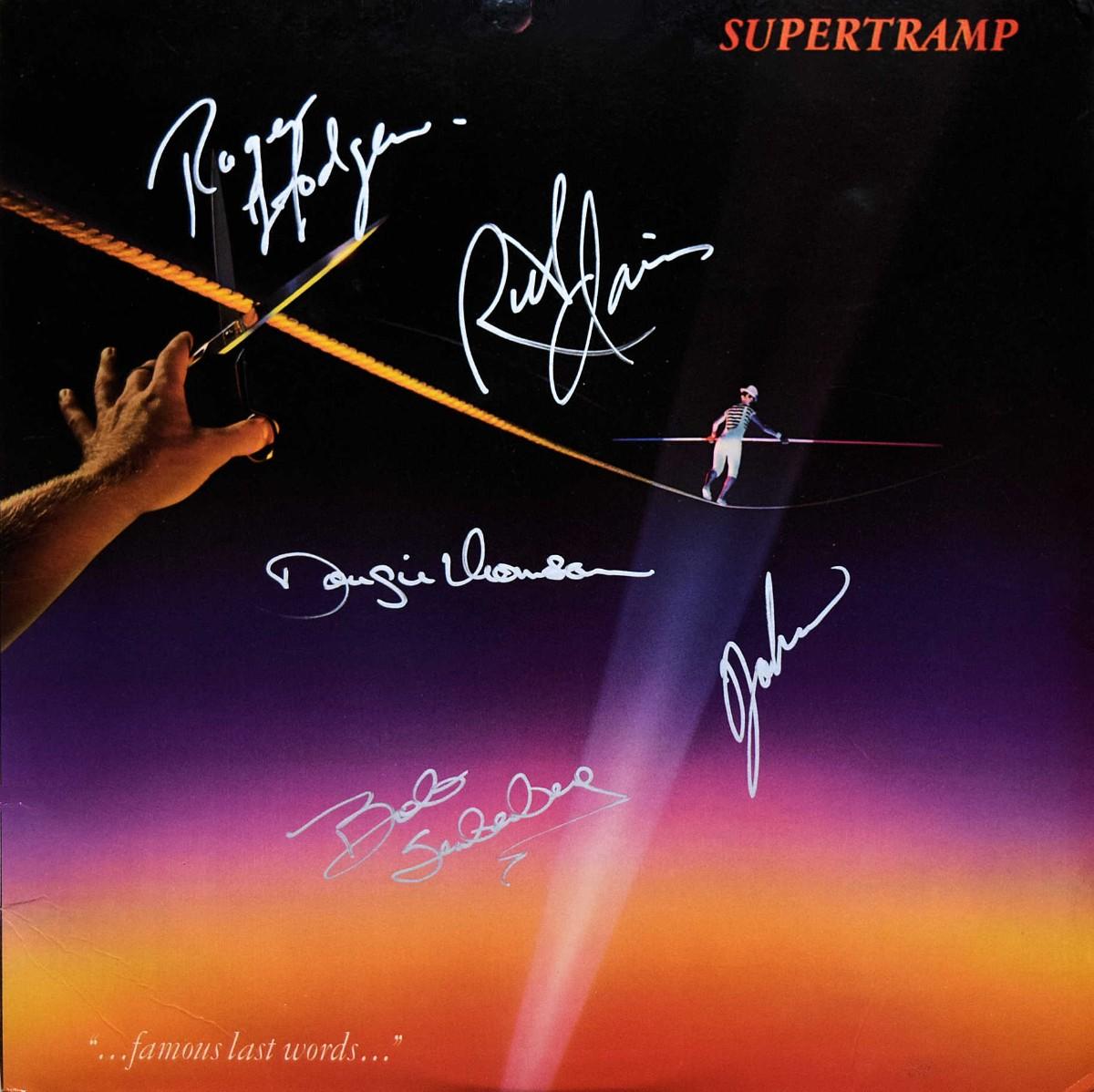This image appears to be the album cover for "Famous Last Words" by Supertramp. It features a dark background that transitions from black at the top to a gradient of purple, pink, yellow, and orange from the middle to the bottom. Dominating the scene is a tightrope that stretches from the upper left corner, dips down towards the center, and rises again to the right. 

A man, dressed in white pants, a black and white striped shirt, and a white hat, balances mid-walk on the tightrope with a long pole in his hands to maintain stability. His back is to the viewer as he moves from left to right, illuminated by a spotlight that shines from below. 

On the left edge, a threatening hand grips a pair of black-handled scissors, poised to cut the rope. Above this dramatic scene, the band's name "Supertramp" is displayed in a reddish-orange font, while the album title "Famous Last Words" appears in white at the bottom, punctuated by ellipses. The cover is further personalized with five signatures from the band members, scrawled in white ink across the image.